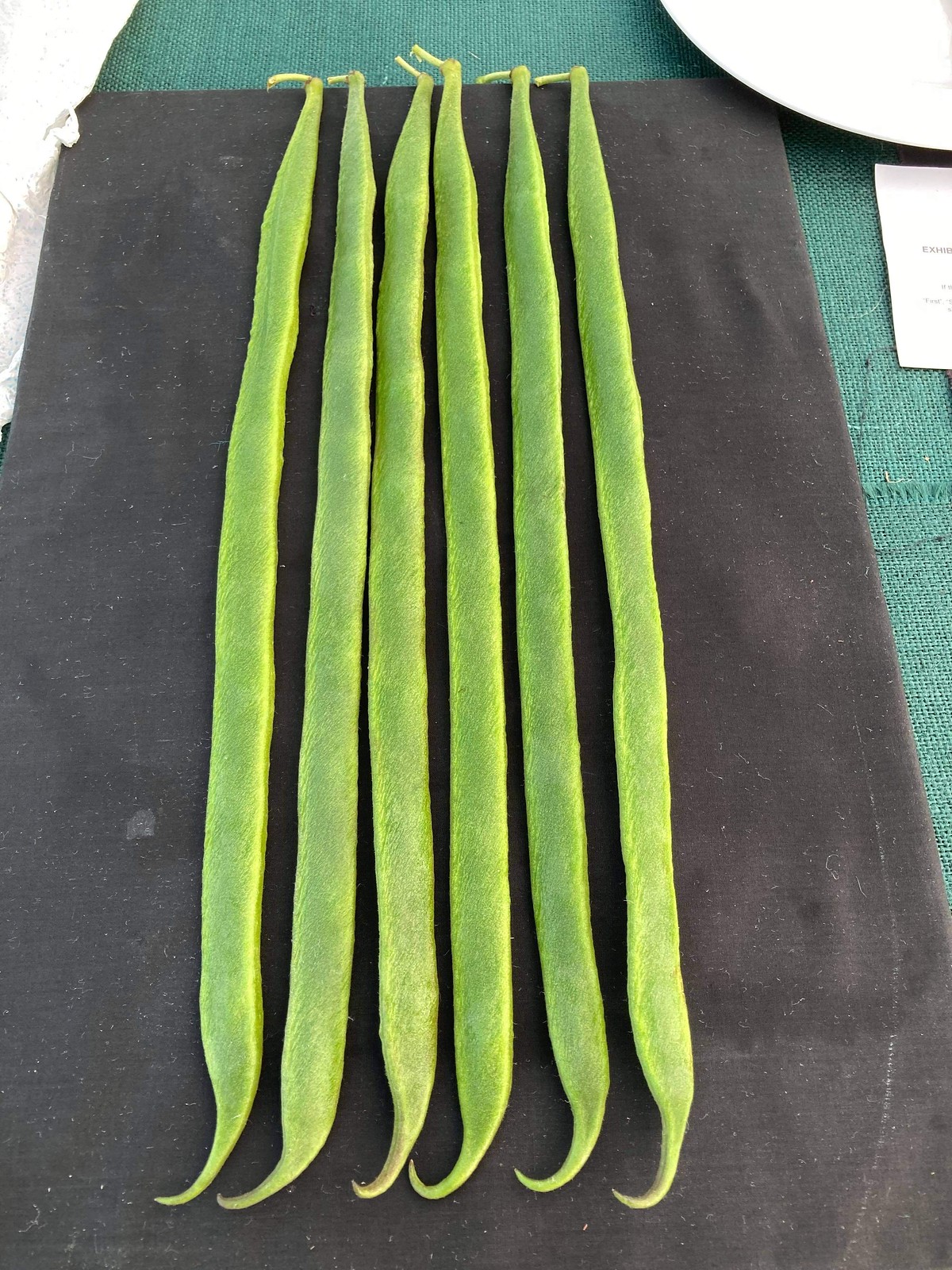This photograph displays six unopened runner beans, each a deep green with subtle yellowish-brown ends. The beans, elongated and slender with noticeable bulges indicating the beans inside, are arranged neatly and side by side along the length of a black cloth, which appears to be placed over a green tabletop or shelf. In the right portion of the frame is a card with some indistinguishable writing, partially out of view, indicating that the setup might be for display or sale. Above the beans, a circular white plate is visible, adding to the arrangement, which appears meticulously prepared. The overall presentation suggests the beans are ready to be prepared for a culinary use, such as in a soup or stew.